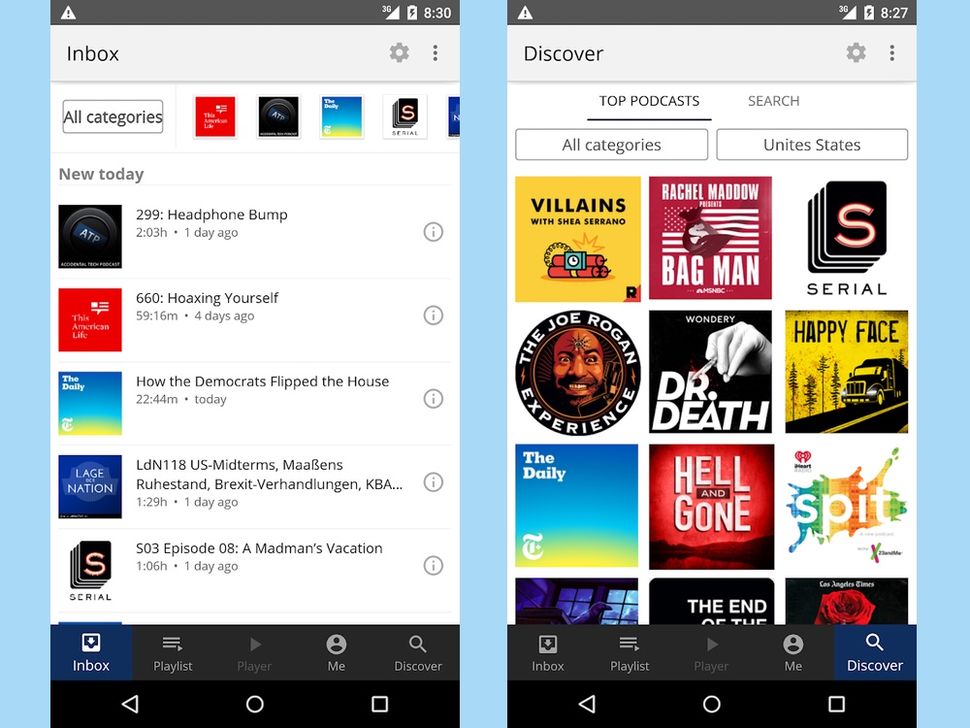The left side of the image displays an inbox, while the right side showcases a "Discover" section with various categories. A pair of headphones priced at $299 and hooks for $260 are listed. Headlines include topics such as "How the Democrats Flip the House", "This is the Nation", and "LDN Woman". Another section mentions recent U.S. returns with phrases like "Mom Ends", "Who Has Stan", "Brexit Burned", and "Logan the KB".

The image also includes icons and listings such as "a129 h1 decal", "Circle Diner", and "Stacks of Cars". Additionally, there is a reference to a serial "s03". A man in medication is depicted along with an inbox, a playlist, and a prayer. The "Discover" section further features a bar on the right, with a top bar that reads "704 battery" and "827". 

Highlighted podcasts include "Feelings with Rachel", "My Dog Batman", "The Joe Rogan Experience", and "Dr. Happy Face". There are also mentions of "Dearly Helen", "God Spit Bucks", and a music playlist. The overall layout seems to be a busy mix of various elements from inbox and discovery sections.